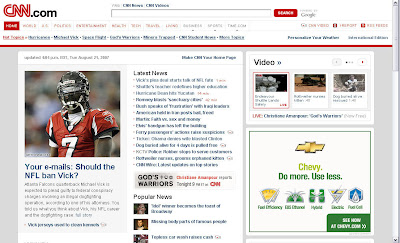The image features a detailed snapshot of the CNN.com homepage. In the upper left-hand corner, the iconic CNN logo is prominently displayed in large red letters. Adjacent to the logo is a search bar with the word "search" to its right, which users can utilize to find specific content on the site. 

Dominating the left side of the page is the main article headline, which reads "Your Emails: Should the NFL ban Vick?" Above this headline is an accompanying picture of the football player Michael Vick, dating back to the period of his notorious dog fighting controversy. 

On the right-hand side, a column titled "Latest News" features multiple story headlines in bold black letters. Further down on the middle right-hand section, there's a highlighted story titled "God's Warriors." 

An advertisement for Chevy is situated to the right of the "God's Warriors" story, bearing the slogan “Do more, use less” alongside the Chevy symbol. Above the ad, three video preview boxes indicate available video content on CNN.com. Although the specific video options are not visible, users can click on any of these boxes to play the corresponding videos.